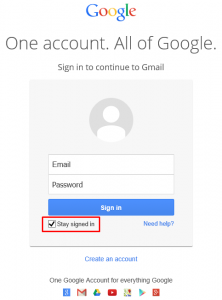The image depicts a blurred and compressed screenshot of a Google sign-in or sign-up page viewed on a smartphone. At the top of the image is the iconic Google logo in its standard colors. Below the logo, the phrase "One account. All of Google." is displayed in gray letters. The text "Sign in to continue to Gmail" appears beneath this line.

The central part of the image shows a generic user profile icon next to two empty fields labeled "Email" and "Password," indicating where users would input their credentials. Below these fields is a light blue button with the word "Sign in" written in white.

A check box in the lower left corner of the button is ticked off, labeled "Stay signed in." This check box is emphasized by a red rectangle. Below the sign-in button, to the right, there's a blue text link that reads "Need help?" accompanied by a question mark.

A thin gray horizontal bar separates this area from a blue text option reading "Create account," centered towards the bottom. Finally, at the very bottom, the text "One Google Account for everything Google" is displayed, along with a series of logos representing various Google services, such as Gmail, Google Drive, YouTube, Google Maps, the Google Play Store, and Google+.

The overall background of the image is plain white, and only the captured part of the phone screen is visible, with no additional browser chrome or icons present.